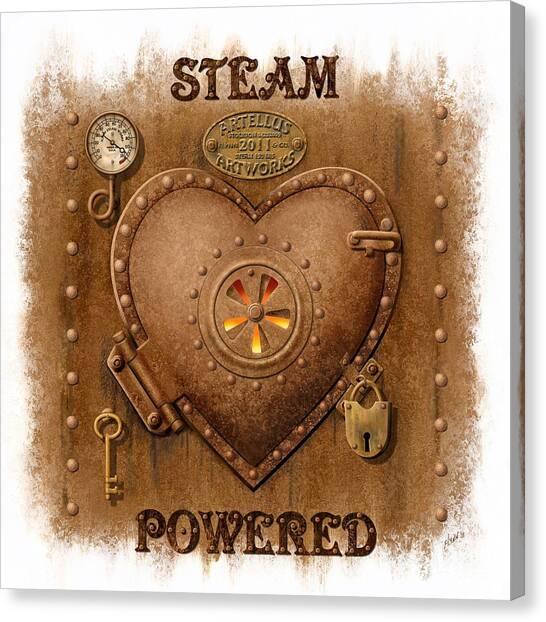The image is a detailed artistic drawing on a canvas transitioning from a white perimeter to a brown center. Central to the composition is a metal heart resembling a component from a steampunk aesthetic, characterized by its deep brown hue and intricate design elements. The heart is hinged and locked, hinting at a functional object, with a handle indicating it can open. The heart features a series of five vent-like openings arranged in a circle through which fiery hues of yellow and orange are visible, suggesting an internal flame or furnace.

Above the heart, the word "STEAM" is prominently displayed in an older, vintage font in a lighter brown color. Beneath "STEAM" is an oval badge labeled "ARTELIS" at the top, "ARTWORKS" at the bottom, and the year "2011" in the center. Hanging from the heart's left side is an old-fashioned key, while a lock, also in brown, secures the heart on the right side. Additionally, on the top left area of the heart, there is a white pressure gauge with black numerals encased in brown metal. Below the heart, the word "POWERED" is inscribed, completing the text "STEAM POWERED." The predominant colors in the artwork include various shades of brown, white, red, yellow, orange, and black, creating a cohesive steampunk theme and positioning the heart as the focal point at the very center of the image.